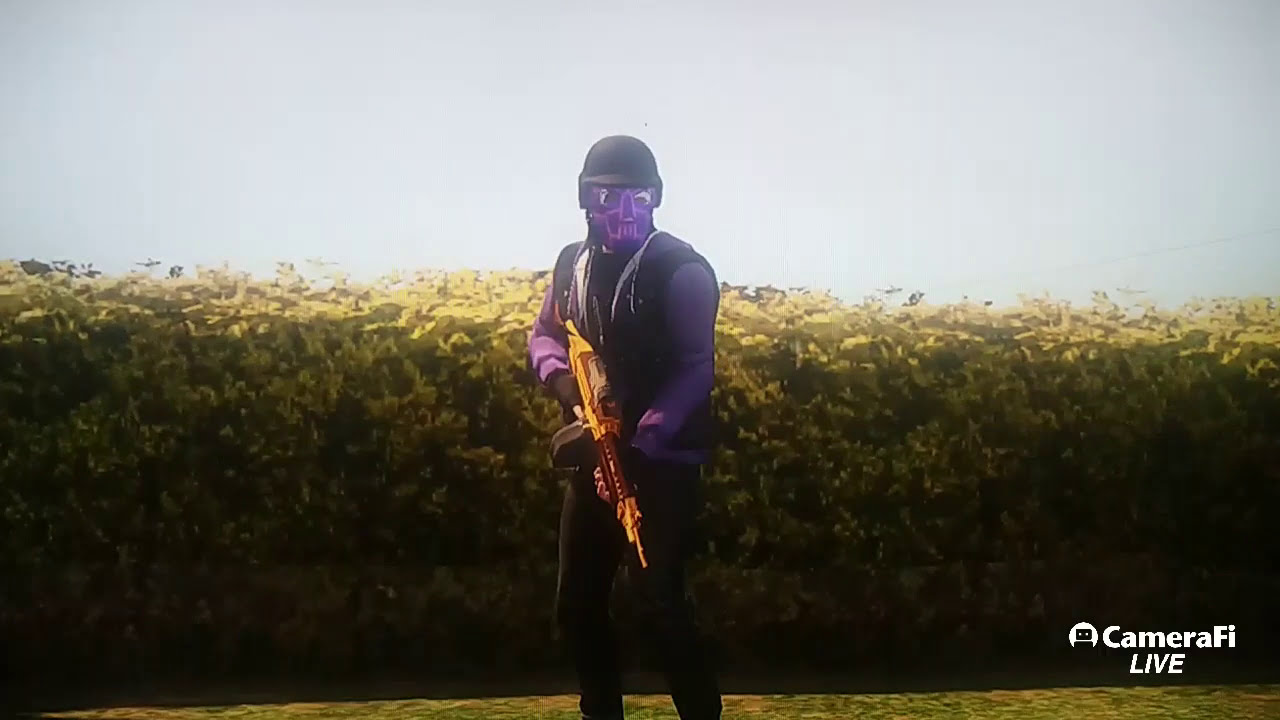The image appears to be a computer-generated scene, potentially a screenshot from a video game or 3D-rendered animation. At the center of the image stands an armed character in paramilitary attire. The character wears a black, rounded helmet reminiscent of a stormtrooper's, paired with a purple mask and a black military-style vest over a long-sleeved dark purple shirt. The ensemble is completed with tight black pants. The character holds a large gun with a black drum barrel and a golden body, which features a reddish hue near the front chamber; the gun is pointed downward. The setting includes a tall green hedge casting shadows at the bottom, with a clear blue sky as the backdrop. The base of the image reveals a partially visible grassy field. White text in the bottom right corner reads "Camera Phi Live" in italics, with "C" and "F" capitalized.